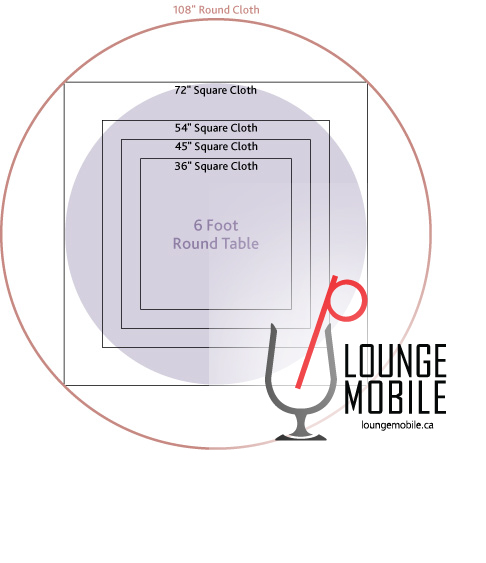This detailed graphic illustration, depicting a tablecloth sizing guide, features a 6-foot round table represented in light purple at its center. Surrounding the table are four black-outlined squares labeled as 36", 45", 54", and 72" respectively. Above the image, a brown-colored circle extending to the edges of the graphic signifies a 108" round cloth, with text noting “108'' round cloth” in the same brown hue. At the bottom right corner, the logo for Lounge Mobile is displayed, featuring a gray glass with a black bottom, a red stirring straw shaped like the letter P, accompanied by black text stating "Lounge Mobile" and "loungemobile.ca." The entire graphic is set against a white background, providing a clear and informative guide for selecting the appropriate tablecloth sizes for a 6-foot round table.